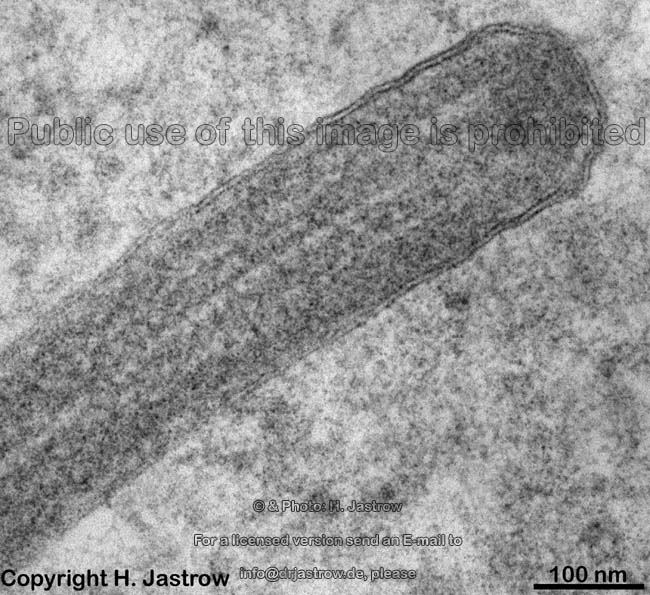This black and white close-up image, which appears to be a microscopic view of a probiotic cell or some type of smear intended for scientific observation, features a distinctive speckled pattern with an arc resembling a rounded driveway or cul-de-sac stretching from the lower left to the upper right of the photo. At the top third of the image, a watermark spans from one side to the other, stating "public use of this image is prohibited." The bottom of the image includes a licensing note directing inquiries to info@drjastro.de, and at the bottom left is the copyright notice "© H. Jastro," both in bold, black font. Additionally, the bottom right corner features a scale labeled "100 nm," indicating a measurement of 100 nanometers.